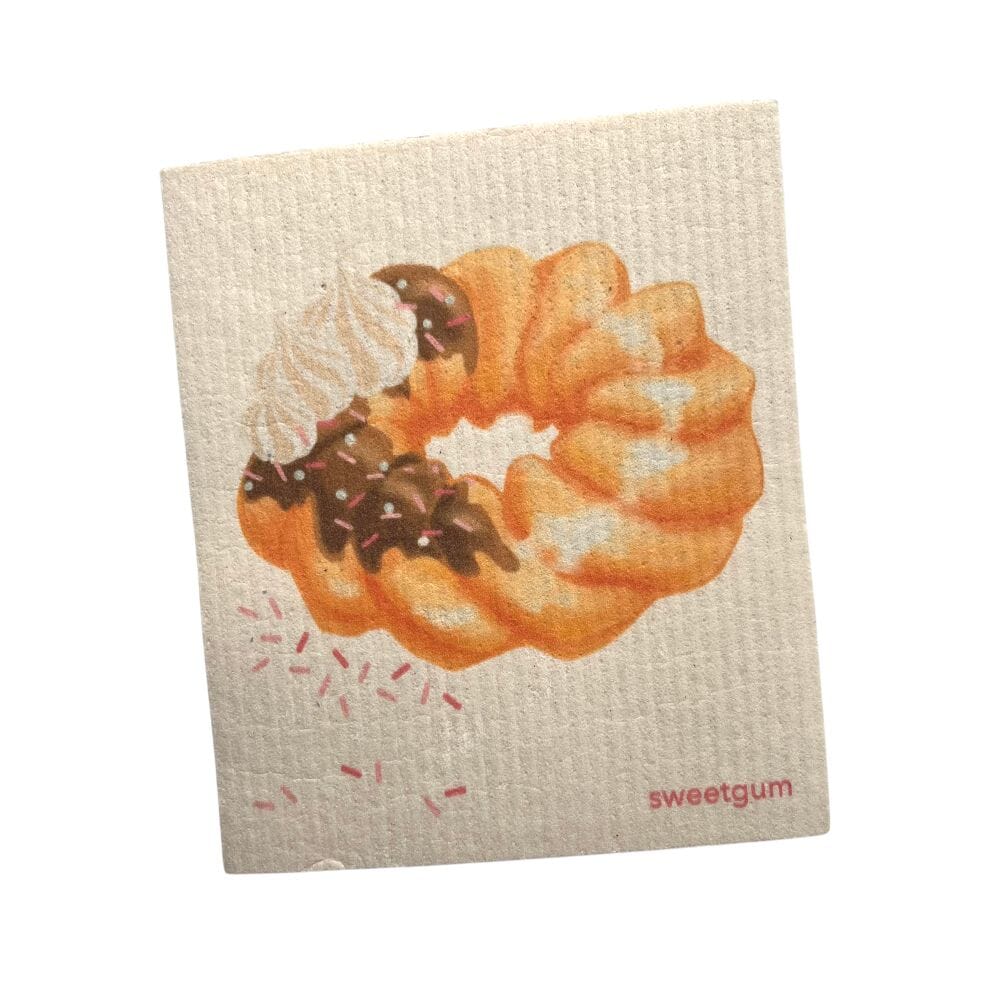This image displays an off-white Swedish dishcloth with a highly detailed and artistic depiction of a cruller donut. The donut is a French cruller style, characterized by its ridged and swirled texture, made from a yellow vanilla cake. It is adorned with chocolate frosting that drips down its sides, and is sprinkled with a mix of small white, pink, and red sprinkles, some of which are depicted falling off the donut. To further embellish it, three small dollops of white whipped cream or meringue are artistically placed on top of the frosting. The background of the dishcloth features a textured, corrugated appearance that mimics parchment paper. In the bottom right corner, the brand name "sweetgum" is printed in pink block letters.